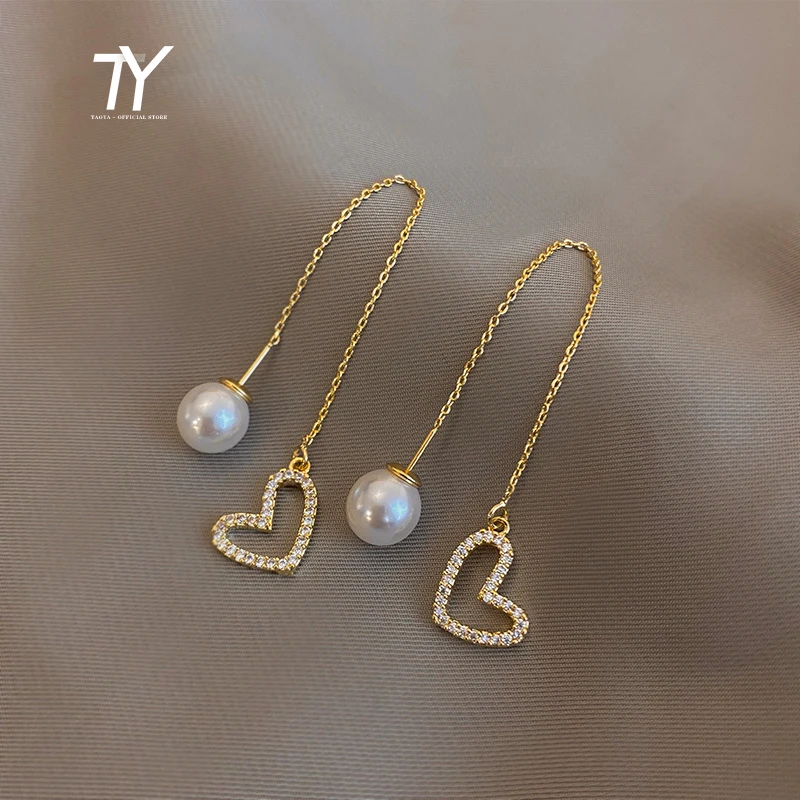In this image, we see two pieces of jewelry, specifically gold chains, displayed on a bunched-up brown or gray cloth material that creates a small hill-like appearance. Each chain forms a narrow, upside-down U shape as they cascade down. The chain on the left features a transparent, pearl-like orb with a gold top, exuding a glossy, reflective surface. On the right chain, a heart-shaped pendant adorned with numerous transparent gems, likely diamonds or crystals, dangles elegantly. In the top left corner of the image, there is a logo consisting of an interlocking T and Y, suggestive of the TY Toyota official store, with some small, unreadable text beneath.